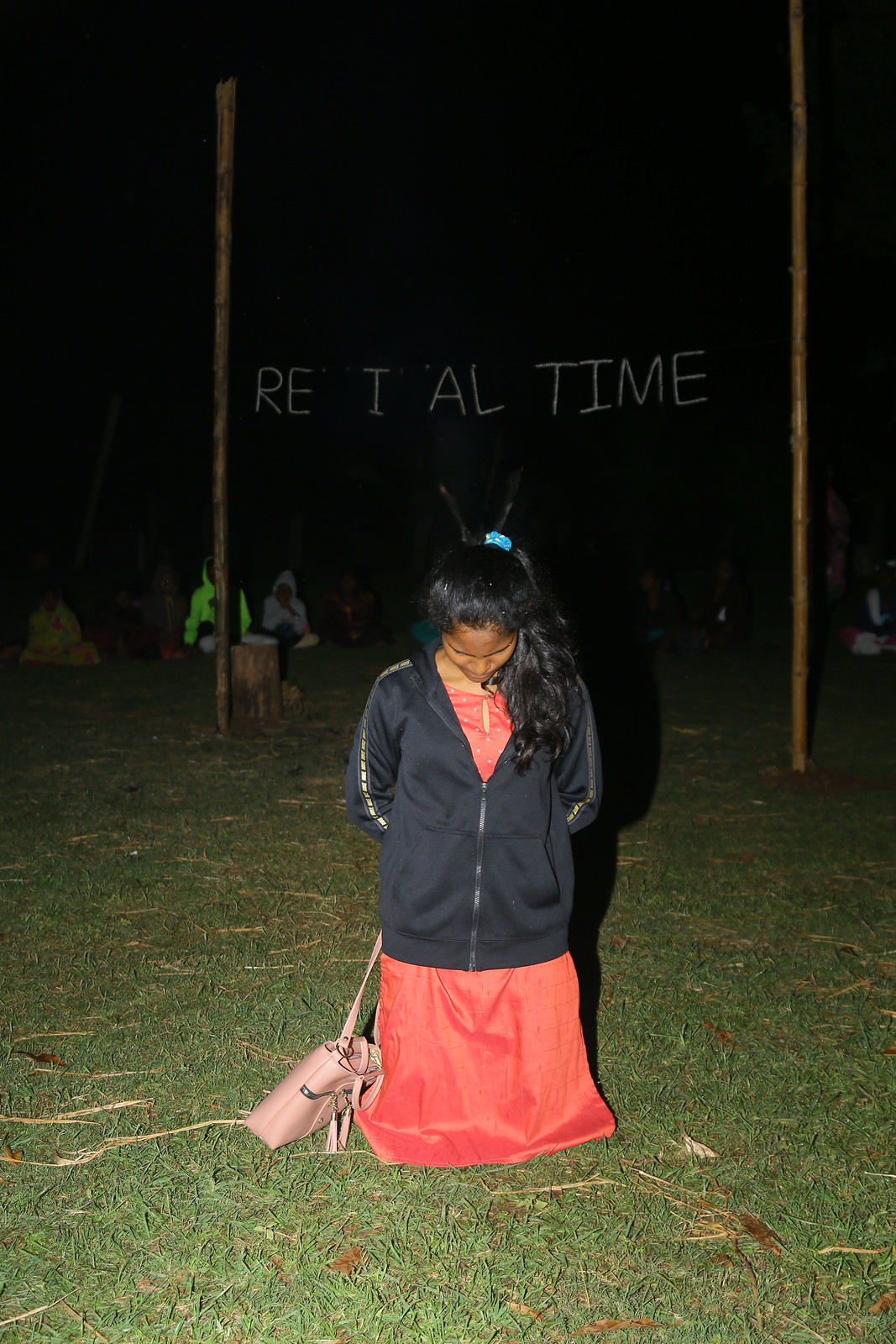In this image, a young woman of Indian descent is centrally positioned kneeling on a grassy area. She has dark skin and long black hair that falls to her chest, tied back with a blue hair tie. She wears a black zip-up windbreaker jacket with yellow stripes along the sleeves, zipped three-fourths of the way over a red polka dot dress. Her hands are behind her back, one holding the strap of a large light pink purse resting on the ground to her right. She appears to be deep in thought, prayer, or meditation with her head bowed. The setting is outdoors at nighttime, relatively dark but with a few individuals distantly visible, sitting on the ground in the background. A sign positioned between two bamboo poles behind her reads "R-E-I-A-L space time," though some letters appear to be missing.